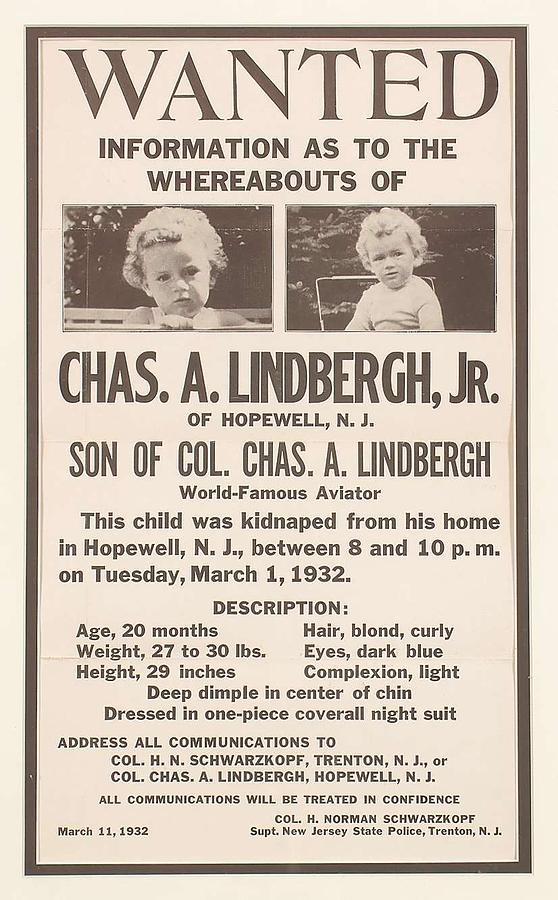This is a black-and-white photograph of a vintage newspaper clipping from the 1930s, showcasing a wanted poster seeking information on the whereabouts of the missing Lindbergh baby. The flyer features a black rectangular border and a predominantly text-based design, with two close-up photographs of the baby positioned in the upper half. The photos depict a white toddler with short, curly blonde hair, seated outdoors—one image showing the child in a wagon and the other in a chair.

The most prominent text at the top reads, in large capital letters, "WANTED INFORMATION AS TO THE WHEREABOUTS OF CHAS. A. LINDBERGH, JR. OF HOPEWELL, NEW JERSEY, SON OF COLONEL CHAS. A. LINDBERGH, WORLD-FAMOUS AVIATOR." Additional information is provided, detailing that the child was kidnapped from his home in Hopewell, New Jersey, between 8 and 10 p.m. on Tuesday, March 1st, 1932. The child's description follows: age 20 months, weight 27 to 30 pounds, height 29 inches, blonde curly hair, dark blue eyes, light complexion, and a deep dimple in the center of his chin. He was dressed in a one-piece coverall night suit at the time of the kidnapping.

The flyer advises that all communications should be addressed to Colonel H. N. Schwarzkopf, Trenton, New Jersey, or Colonel Chas. A. Lindbergh, Hopewell, New Jersey. All communications will be treated in confidence. The poster is dated March 11th, 1932, and lists Colonel H. Norman Schwarzkopf, Superintendent, New Jersey State Police, Trenton, New Jersey, in the bottom right corner.